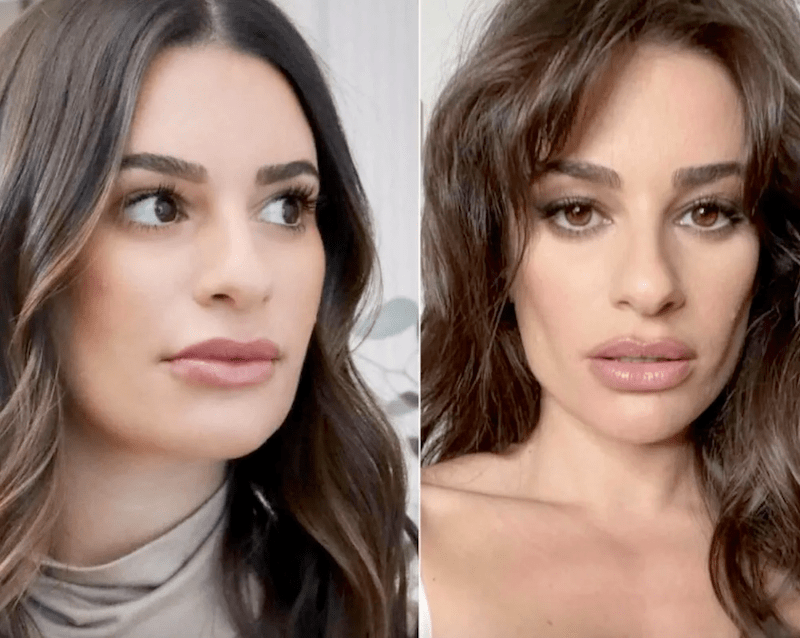This image is a split-screen collage featuring two side-by-side photographs of the same female actress, potentially named Leah. On the left, she is seen with natural, full cheeks, larger eyes, and average-sized lips, wearing a grey turtleneck. Her long brunette hair cascades in soft waves with subtle highlights. She is looking towards the right into the distance with a serene expression. In contrast, the right side presents her with more pronounced cheekbones and fuller lips, suggesting cosmetic enhancements. Her hair appears curlier and messier, giving it a fuller body. In this image, she is looking directly at the camera with sultry and dark makeup, and she appears to be unclothed. The before-and-after effect highlights noticeable changes in her facial structure and overall appearance, lending an impression of increased age in the second image.